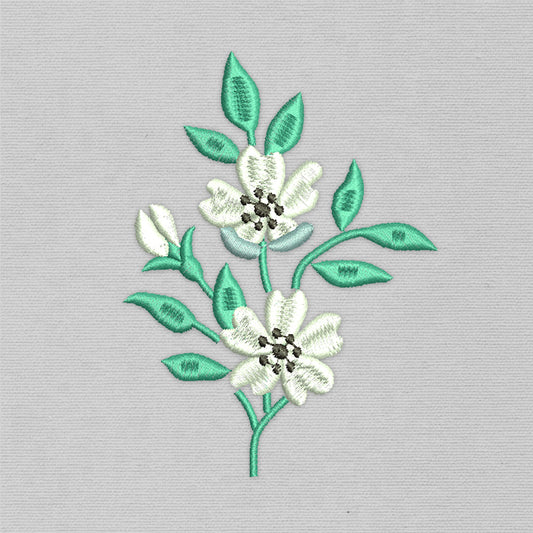This image showcases a detailed embroidery of a flowering plant, meticulously crafted onto a light green cloth. The central design features a plant with lush green leaves and a green stem. Two white flowers with five petals each are prominently displayed, each boasting a brown central area. A third flower, yet to fully bloom, can be seen on the left side. Contrasting the green fabric, the intricate embroidery appears almost as if painted, offering a beautifully natural depiction. The overall artwork is framed within a square shape, enhancing its presentation. This piece combines elements of white, green, and earthy browns to create a visually appealing and ornate floral design.